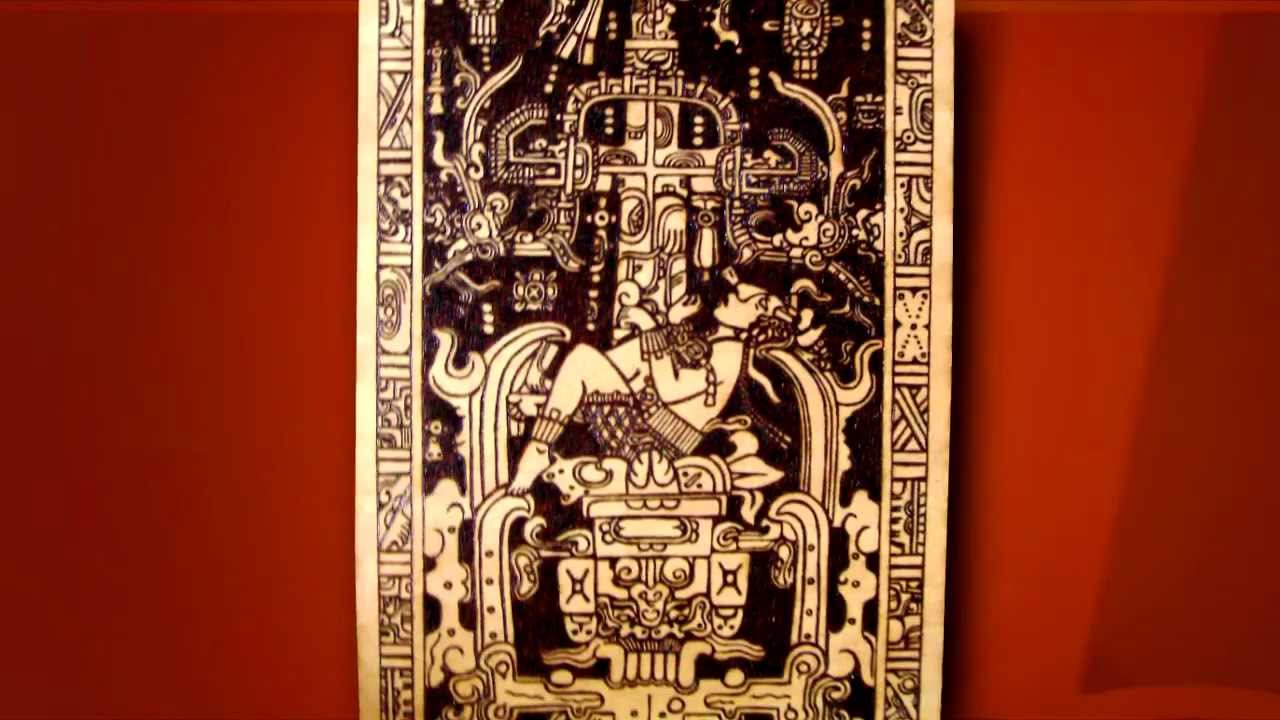This image features a piece of intricate black and white artwork centered on a vertical rectangular tile or panel. The backdrop is a bold red wall, casting a triangular shadow on the right. The artwork itself, framed in gold, appears to depict an elaborate scene with a man, possibly of Mayan or Indian descent, sitting on a detailed throne or altar. The man is facing left, with his knees bent towards his chest and hands in the air, suggesting a ritualistic or sacrificial context. Surrounding the figure are various ornate designs, including squiggly, square, and X-shaped lines. Additionally, a series of vertical rectangles with intricate patterns run along the edges of the artwork, enhancing its complex and ceremonial aesthetic.